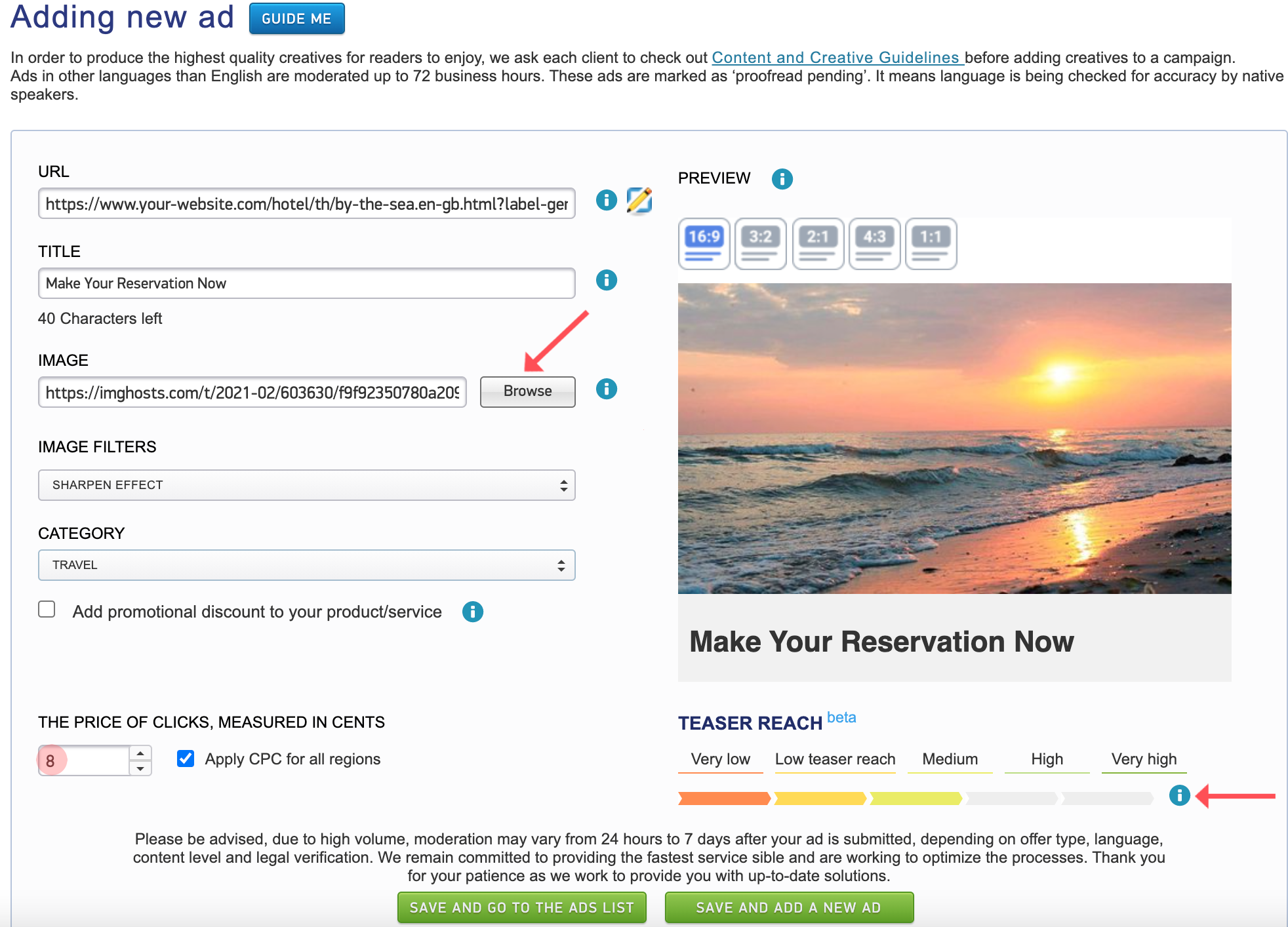**Detailed Screenshot Description:**

The image depicts a desktop screenshot of an unidentified website, where the browser type, web address, and operating system are not visible. 

**Top Section:**
- At the upper left corner, the text "Adding New Ad" is prominently displayed in dark to medium blue print.
- Adjacent to this is a medium blue square button with white text that reads "Guide Me".

**Instructions and Guidelines:**
- Below the title, there is a paragraph emphasizing the importance of producing high-quality creatives. It urges clients to review the hyperlinked "content and creative guidelines" before adding creatives to a campaign.
- It mentions that ads written in languages other than English are subjected to moderation, which can take up to 72 business hours. These ads are flagged as "proofreading pending," indicating that native speakers are verifying the language for accuracy.

**Ad Details Section:**
- The form field labeled "URL" contains an example link: 
  `https://www.your-website.com/hotel/th/by-the-c.en-gb.html?label-ger`.
- Another form field labeled "Title" has the content "Make your reservation now," with an indicator noting that there are 40 characters remaining. Each section has a small info icon for additional details.

**Image and Filters:**
- There is a red arrow pointing to an option for browsing and selecting images.
- An image filter drop-down menu shows the option "Sharpened Effect".
- A category drop-down menu is visible, displaying the "Travel" category.

**Promotional and Pricing Options:**
- There’s an unchecked checkbox labeled "Add promotional discount to your product/service".
- Below it, a field marked "Price of clicks measured in cents" shows the value "8," which appears to be highlighted in red, suggesting it can be adjusted.
- A checked blue checkbox labeled "Apply CPC for all regions" is present.

**Image Preview and Teaser Reach:**
- Ad formats for previewing the image include options such as 16:9, 3:2, 2:1, 4:3, and 1:1.
- An image of a sunrise or sunset at a beach is part of the current ad, accompanied by the phrase "Make your reservation now".
- The teaser reach section is in beta, offering selectable options: "Very Low" (in red), "Low" (in orange), "Medium" (yellow-green), "High" (partially visible), and "Very High".
- Another red arrow points to a blue information icon.

**Additional Information:**
- A caution note states that due to high volume, moderation can vary from 24 hours to 7 days after the ad submission, contingent on the offer type, language, content, and legal verification.
- The site expresses a commitment to providing the fastest possible service while optimizing processes. A thank you note is included for patience during these optimizations.

**Action Buttons:**
- At the bottom are two green rectangular buttons with white text: "Save and go to the ads list" on the left and "Save and add a new ad" on the right.

This comprehensive overview suggests that the screenshot belongs to an online ad management platform, designed to help users create, submit, and monitor internet advertisements.